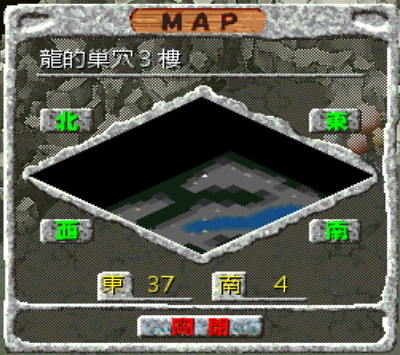This image features a central large square prominently bordered in gray. The central area of the square predominantly showcases an intricate map. At the top center of the image, a brown wooden texture emerges, featuring the word "MAP" inscribed in dark letters. Below this, a series of Asian characters are visible above a long white line. The predominant color scheme of the map is various shades of gray.

In the bottom left corner, a smaller square is present and flanked by green text on its right side. Additional smaller squares can be observed in the bottom left and bottom right sections of the image, interspersed with green, gray, and darker gray hues. The central large square map includes a notable black expanse, sporadically interspersed with light, dark, and medium gray areas, and a section of blue representing a body of water.

Towards the bottom of the map, the numbers 37 and 4 are visible. Near the bottom, there is also an area containing red text. The entire composition is punctuated with various colors and textures, creating a complex and detailed map-like image.